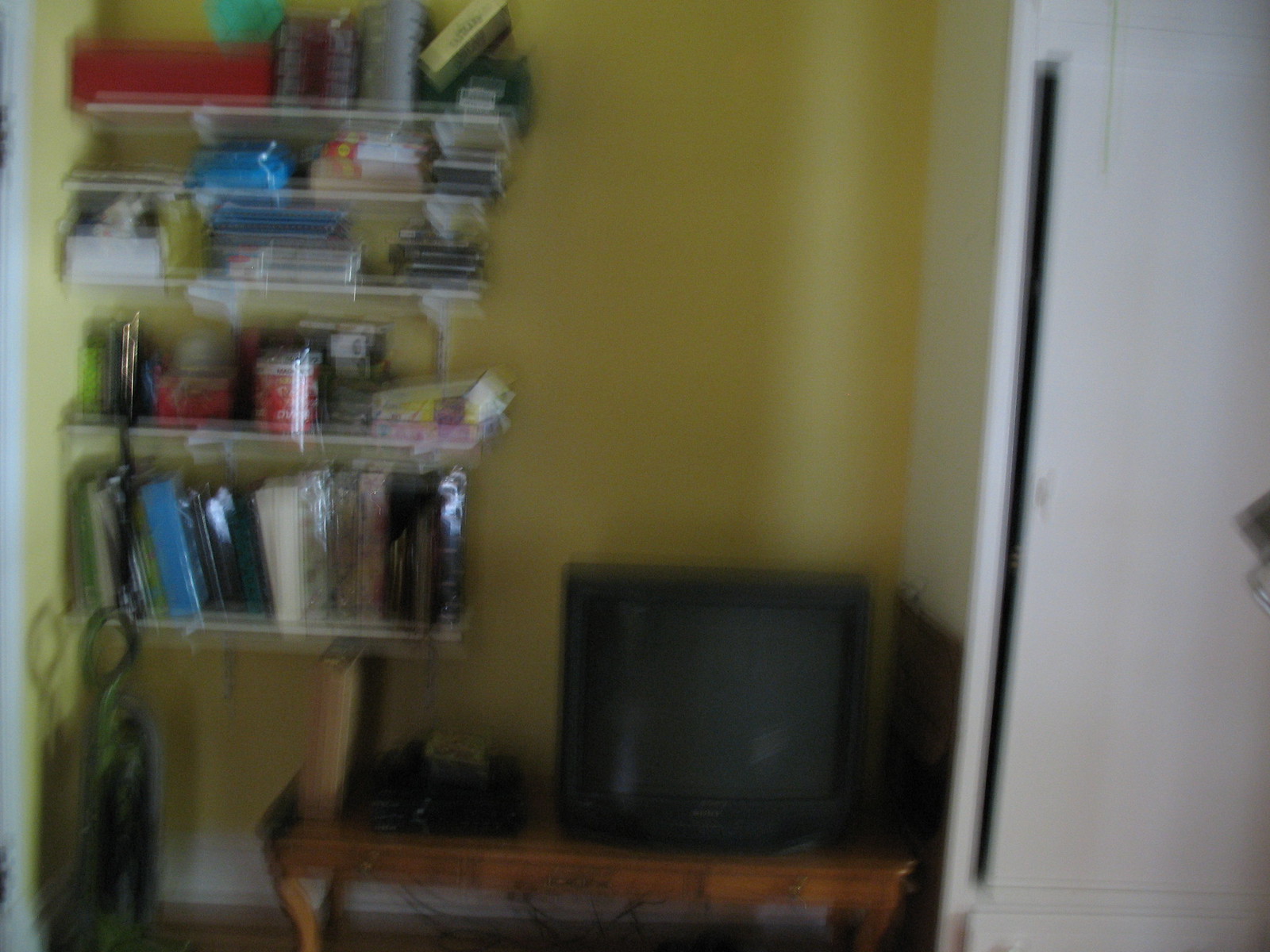This photograph depicts a cluttered corner of a home interior, possibly serving as a storage area within a bedroom, foyer, hallway, or home office. The image is notably out of focus, but several details are discernible. There are multiple shelves, each laden with various items. On the second shelf from the top, round spindle containers hold what appear to be CDRs or DVDRs. The shelves also contain photo albums, spiral notebooks, and various office supplies, including both dry and office goods. Atop the shelves, there are several boxes.

In the lower left corner, a blurred upright vacuum cleaner stands on the floor, next to a small, low mahogany table. An old-fashioned television, complete with a vacuum tube, is positioned in the central lower part of the image. To the right of the television, there is a vertical white closet door. The background wall sports a yellow-green color, adding to the eclectic ambiance of the space.